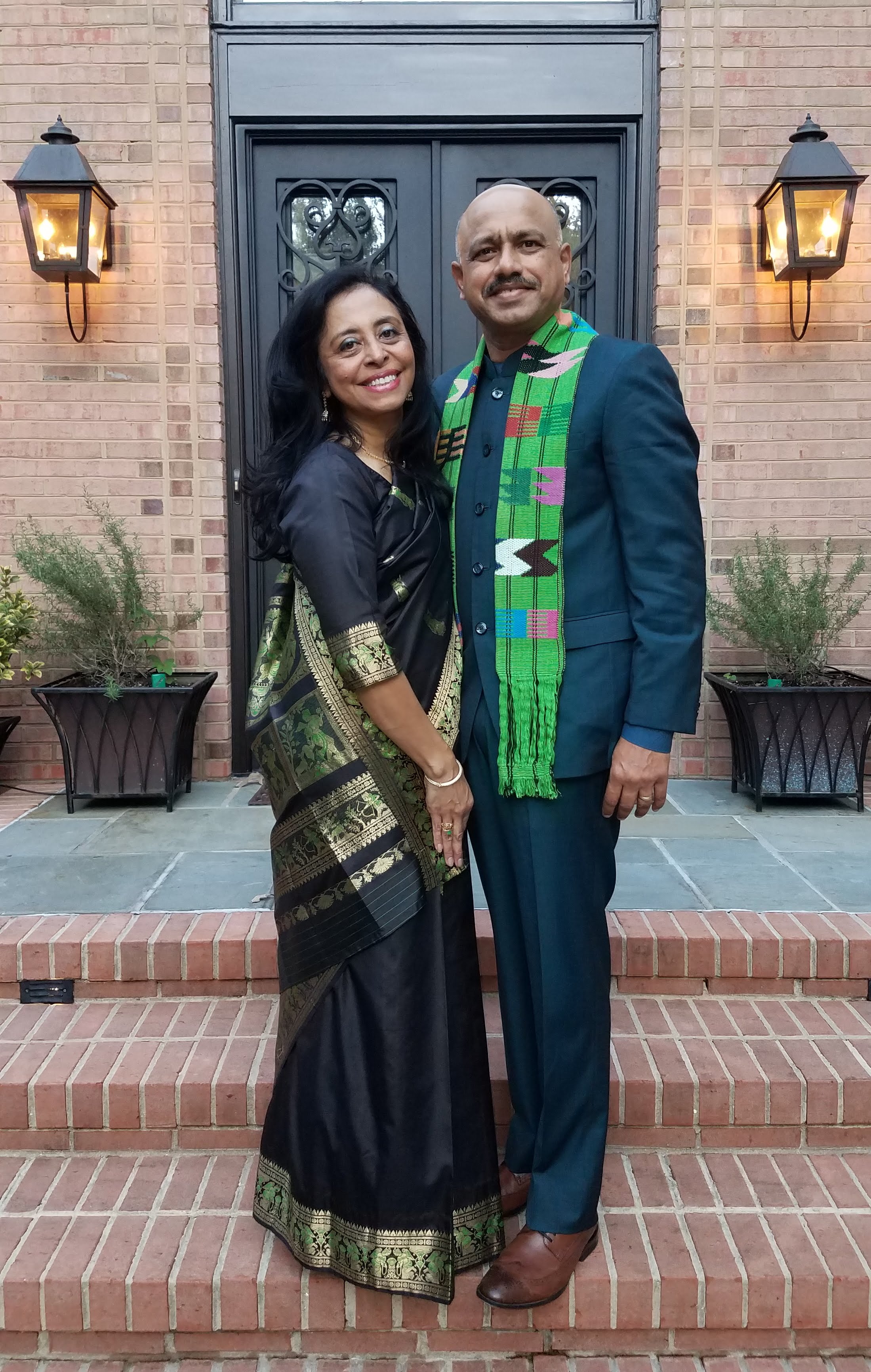In the photograph, a couple, possibly from India or Pakistan, stands smiling on the doorstep of their brown brick house with a prominent double-door entrance adorned with glass panes featuring black metal filigree. The house is flanked by black planters with green foliage and illuminated by porch lights on either side of the door, which sits atop three red brick steps.

The woman, positioned on the left, has long, dark black hair and wears an elegant, very dark blue (almost black) traditional Indian dress made from shiny material. This dress is detailed with intricate gold embroidery and a touch of green, wrapping over her left shoulder like a back smock. She accessorizes with a gold bracelet and a green ring.

The man to her right is bald with a mustache. He is dressed in a dark navy blue suit that buttons up to the neck, complemented by blue dress pants and brown shoes. Around his neck, he drapes a colorful scarf predominantly lime green with blue, pink, black, and white zigzag patterns. Together, they stand proudly in front of their home, radiating warmth and cultural elegance.